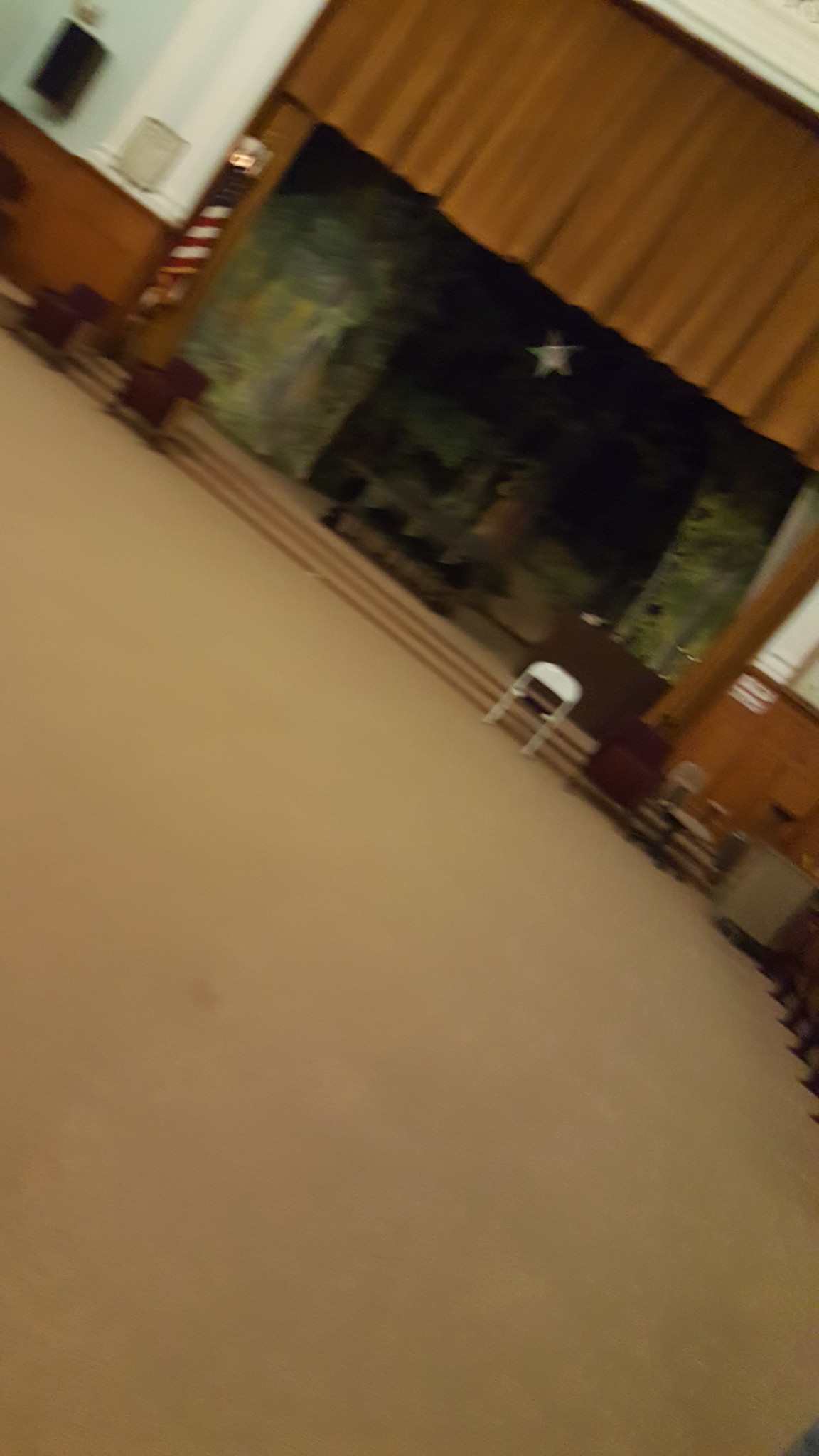This photograph captures the interior of a spacious hall, revealing an expansive room characterized by an abundance of brown carpeting. The rectangular image is slightly blurry and out of focus, adding a sense of mystery and movement. The composition is at a skewed angle, making the room appear as if it is leaning sideways.

In the background, a prominent stage is visible, draped with a large curtain. To the right of the stage stands an American flag, signifying a setting of national or civic importance. At the forefront of the stage, short steps lead up to a solitary white folding chair, indicating a spot for speakers or performers. The image's perspective and the detail of the furnishings create a sense of anticipation, as if the room awaits a gathering or event to begin.